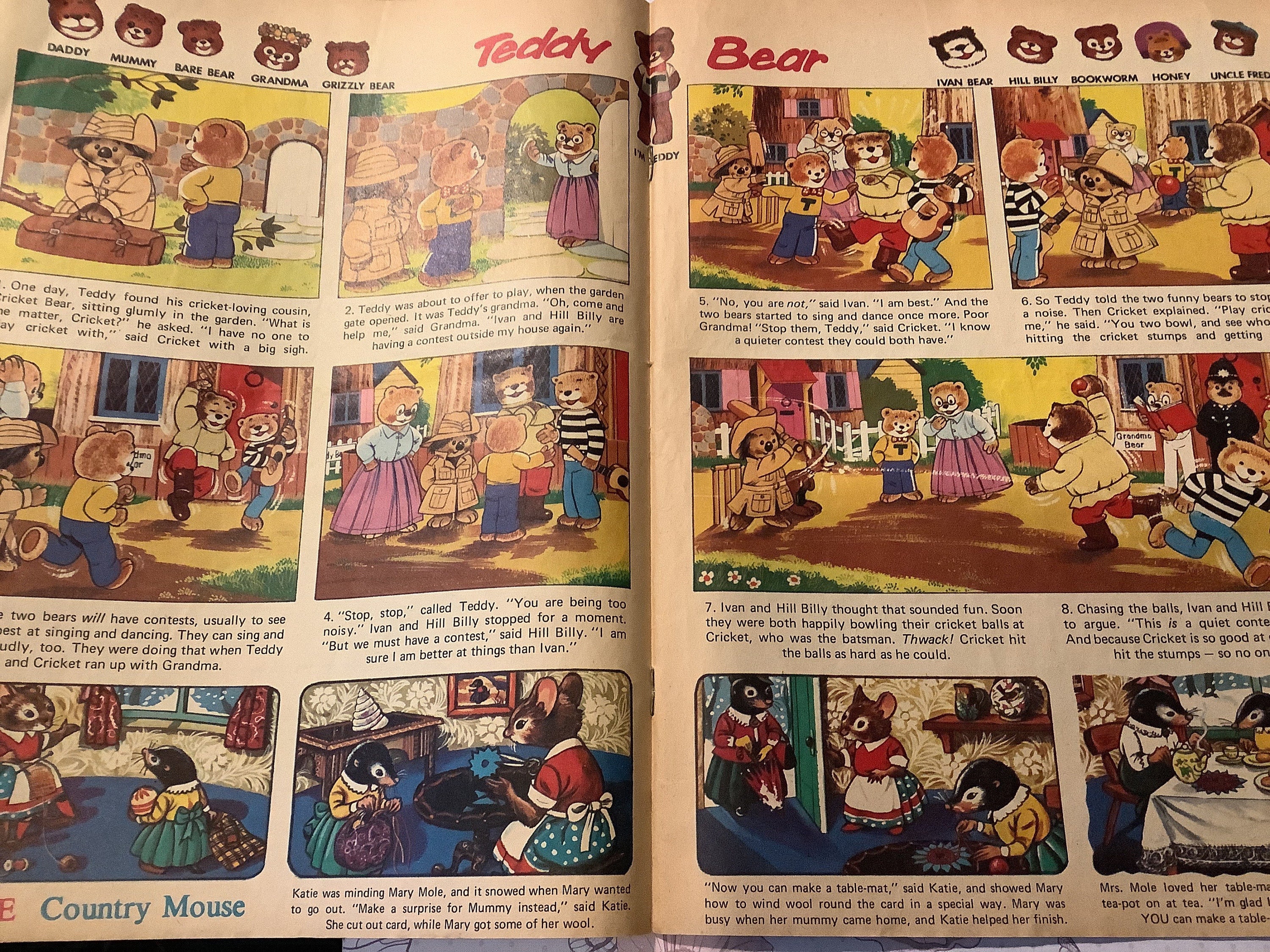This is a rectangular landscape photograph showcasing an open children's book. At the top center of the book, the heading reads "Teddy Bear," accompanied by an illustration of a teddy bear. Along the top edge of the pages, there are five drawings of bear faces, adding a playful touch to the layout. Each page of the book is divided into six quadrants, arranged in three rows from top to bottom and two columns from left to right.

Each quadrant features a distinct illustration, depicting a variety of characters including bears, a mouse, and a skunk. Beneath each illustration, there are descriptive words, likely intended to aid in reading comprehension or vocabulary development for young readers. The vibrant and detailed artwork aims to engage children’s imagination, making the book both educational and entertaining.